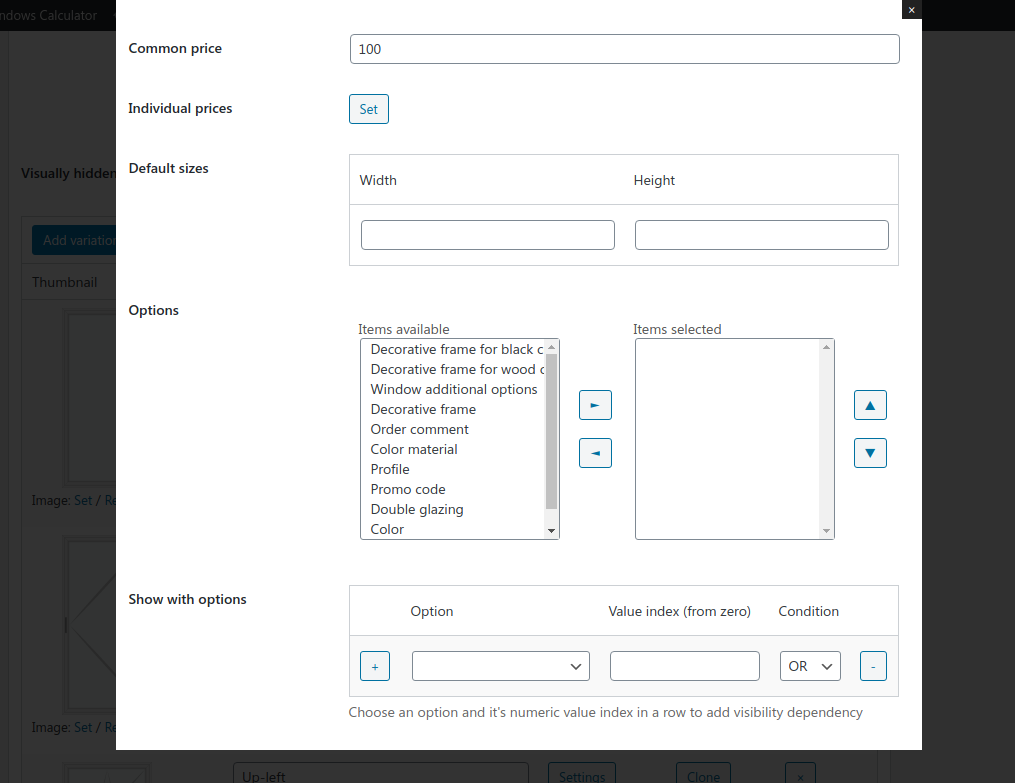In the foreground, a pop-up window dominates the scene with a clean white background. Within this pop-up, multiple fields and settings are visible. At the top, a field labeled "Common Price" is set to 100. Below this, individual price fields are displayed along with a "Set" button. Default size settings for both width and height are present but remain unentered. Additionally, an "Options" section features a dropdown menu and two fields: "Items Available" and "Items Selected," which allow for item swapping. The bottom section of the pop-up reads "Show with options," inviting the user to add various options as needed. On the right side of the pop-up, there is a logic section that allows for combining statements using "AND" and "OR" functions.

In the background, barely discernible text and elements are subtly visible, suggesting a dimly lit area. Words like "add," "thumbnail," and "image" can be faintly made out, scattered sparsely along the edges of the screen. While the background remains enigmatic and hard to make out clearly, its presence hints at underlying complexities within the larger site context.